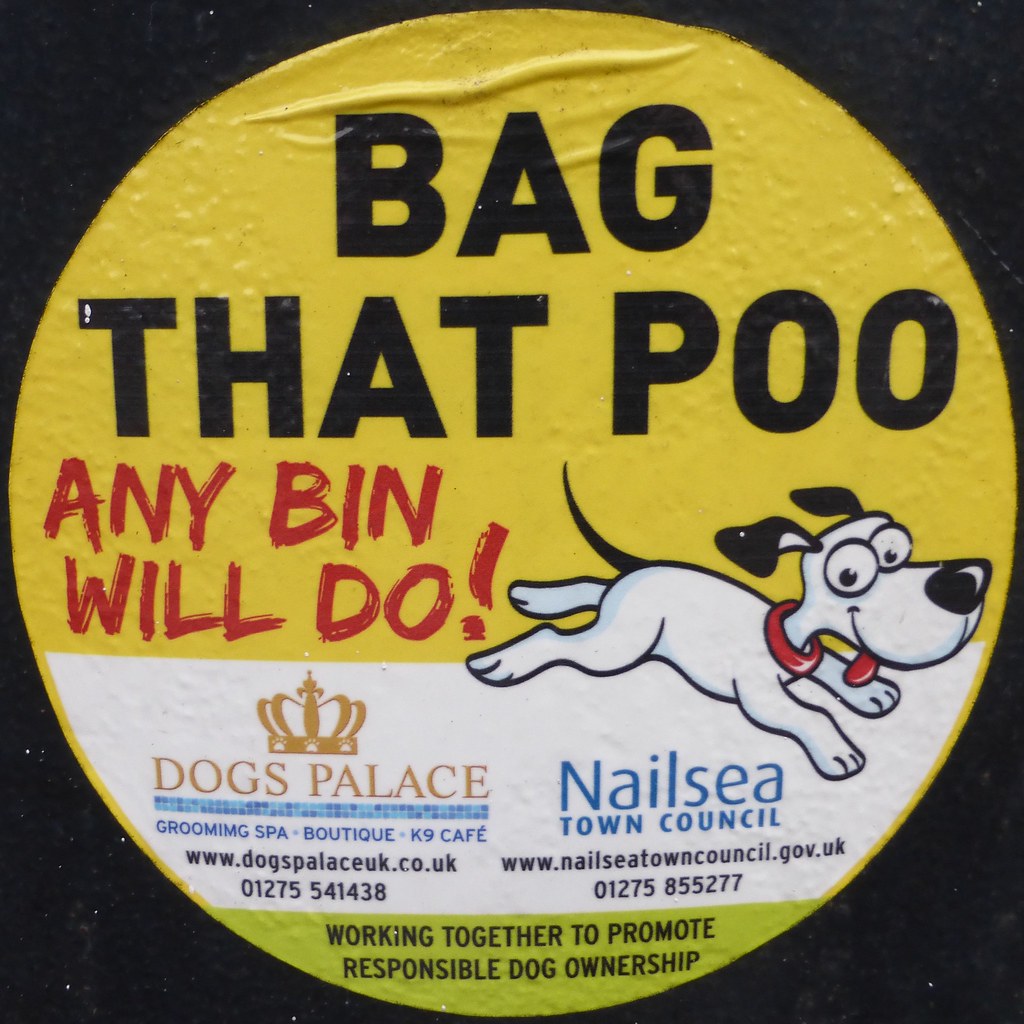The image features a bright yellow sticker set against a black background. At the center of the sticker, bold black text emphatically reads, "Bag That Poo." Located at the bottom left of the sticker, in smaller black text, it states, "Any Bin Will Do." Accompanying the text is an endearing cartoon illustration of a white dog with its tongue playfully sticking out.

Towards the bottom left of the sticker, details about a dog grooming establishment are provided: "Dogs Palace Grooming Spa Boutique Canine Cafe" followed by their website, "www.dogspalaceuk.co.uk," and the contact number, "01275 541438."

On the right side, the sticker includes information about a local governing body: "Nailsea Town Council," along with their website, "www.nailseatowncouncil.gov.uk," and the contact number, "01275 855277."

Encircling the bottom of this yellow sticker, in matching yellow text, the message concludes with, "Working Together To Promote Responsible Dog Ownership." This emphasizes the collaborative effort towards encouraging responsible pet care within the community.